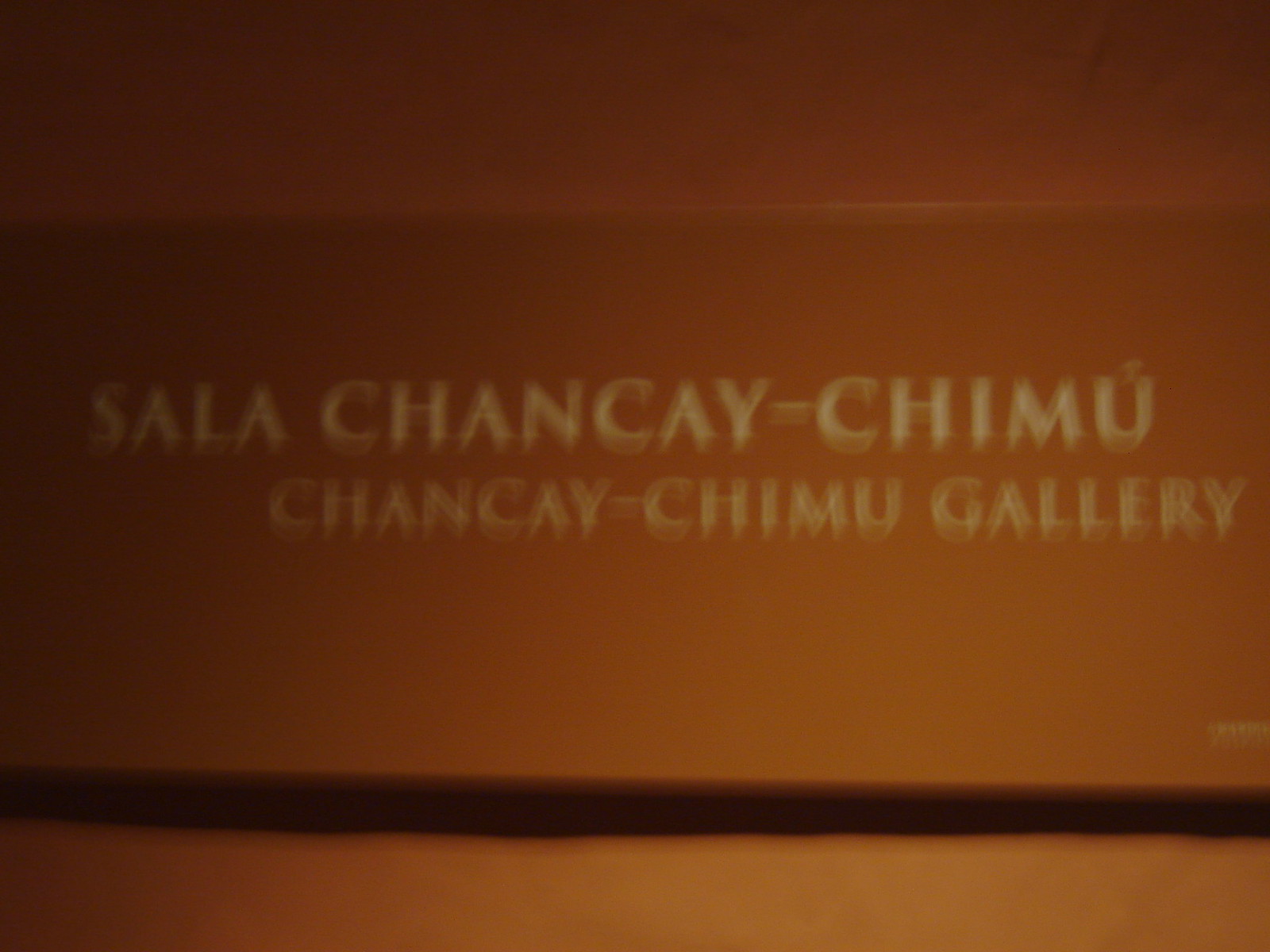The image depicts a sign for the "Sala Chankye-Chimu Gallery." The sign features light-colored text on a predominantly brown background that transitions from darker to a reddish-brown hue, becoming lighter as it goes down. The text, which appears in a fancy, all-caps Roman-style font, is clearly legible despite the image being blurry and low resolution. The sign's writing is centered about midway down the sign and is separated by a solid black line from a darker area below. Intense shadowing is evident between the sign and the wall behind it, adding a notable contrast that emphasizes the simplicity and elegance of the text against the plain, painted wall backdrop.